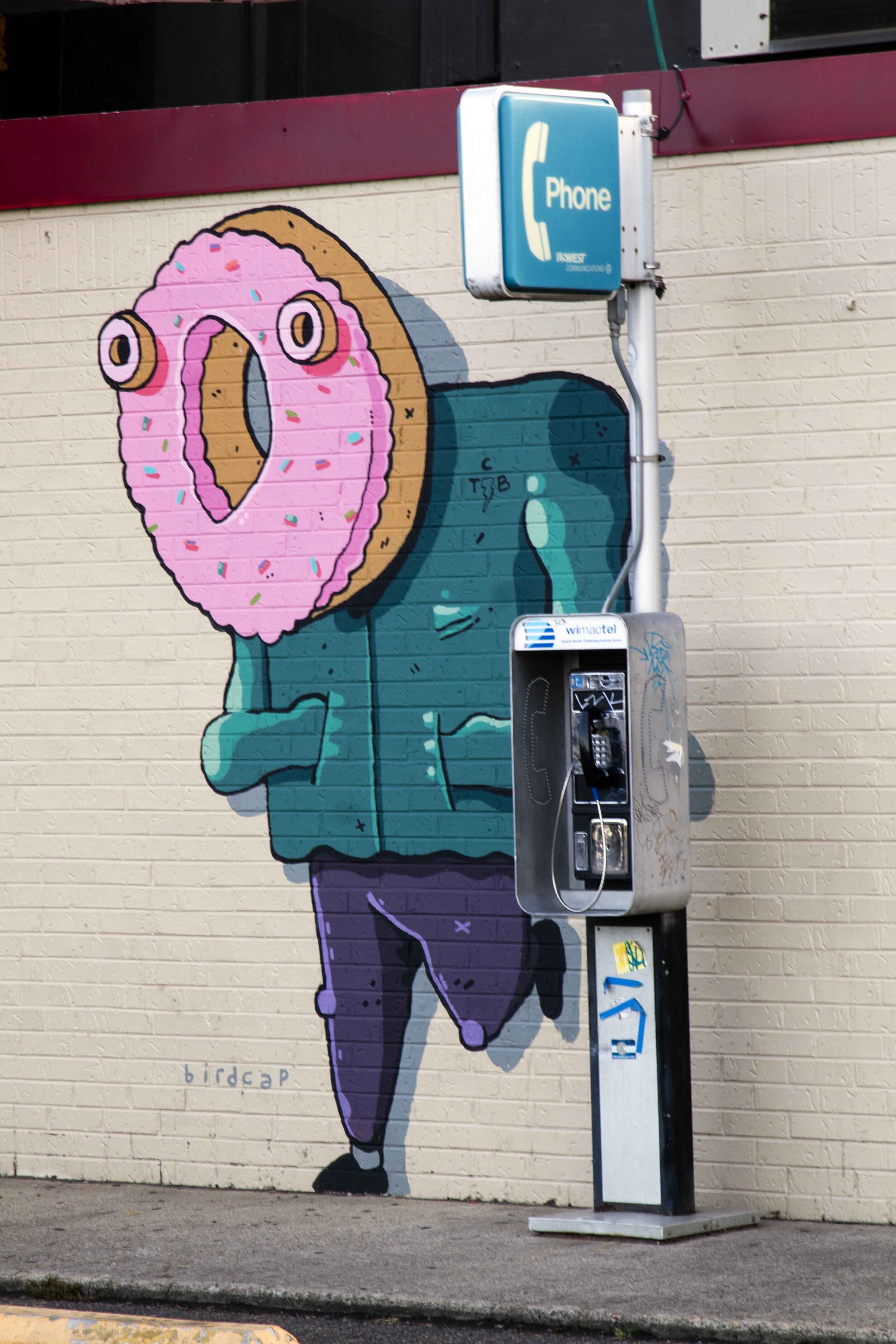The image depicts a realistic outdoor scene captured in a vertical rectangle photograph. The background features an off-white brick wall, approximately eight feet tall, adorned with a burgundy trim at the top and some black material extending upwards. A dark gray sidewalk runs along the base of the wall. On the right side of the image stands a telephone box with a vertical metal pole, displaying a blue sign that reads "phone" in white letters. Next to the telephone box, colorful graffiti showcases a cartoonish, human-like figure with a donut head. The donut head is a large brown ring with pink frosting and sprinkles, with two smaller donuts serving as eyes. The character is dressed in a green, boxy jacket, with its arms tucked into the pockets, blue pants, and black shoes, one of which is propped against the wall. To the left of the graffiti, the words "bird cap" are painted in blue letters.